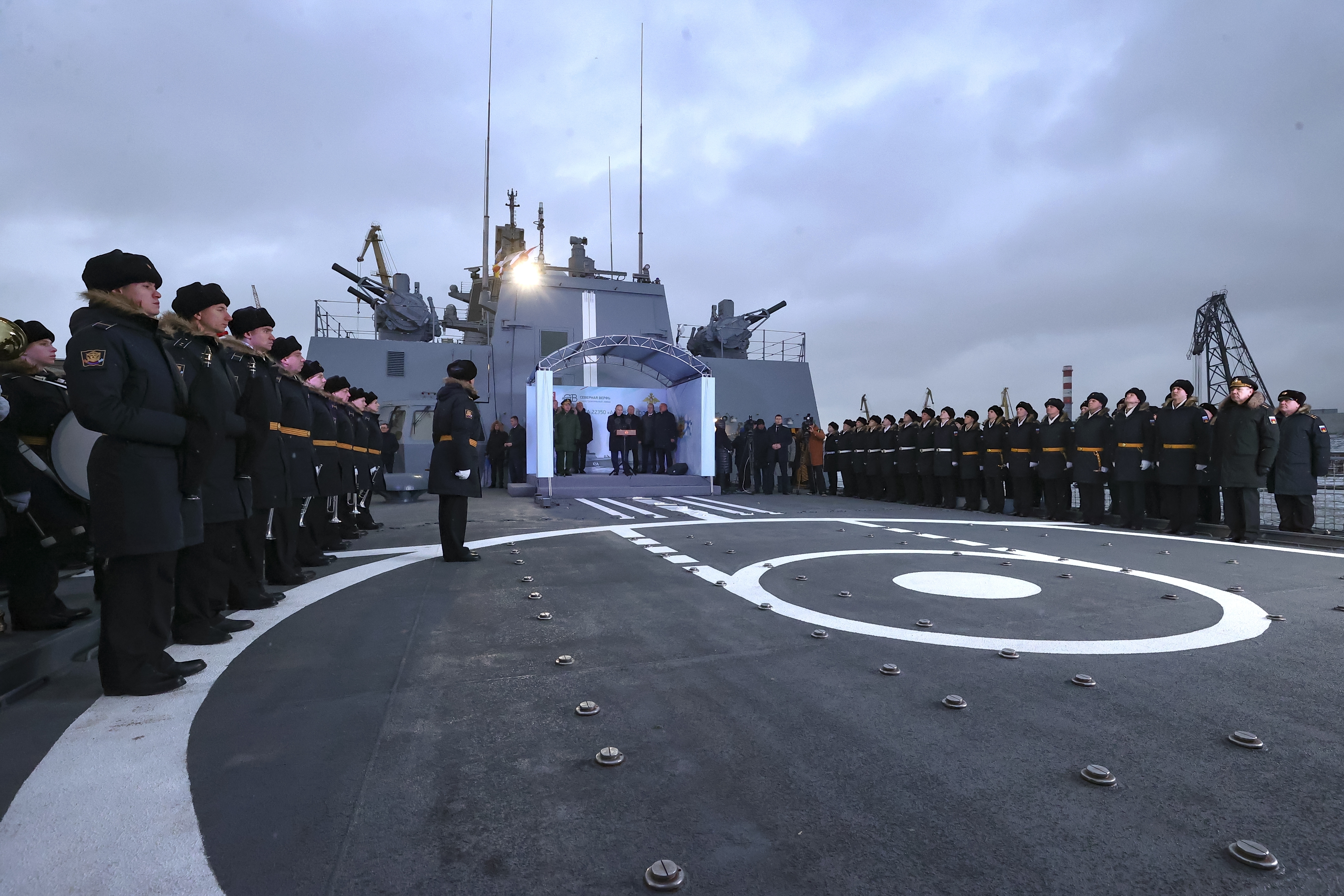The image depicts the deck of a large, gray warship, likely an aircraft carrier or battleship, with features resembling a helicopter landing pad. The expansive, flat surface of the deck is adorned with asphalt-like material, white circular markings, and several dotted lines that lead from the central circle to the left.

Detailed and orderly, the scene is marked by two distinct rows of uniformed soldiers standing on either side of the deck. On the left, the soldiers, attired in long black peacoats with fur collars and black hats, are aligned in rows. Some of these soldiers are distinguished by yellow belts, while those positioned further back wear white belts. A lone officer, facing right, stands out in front of this formation, which resembles a military band, each holding a trumpet. 

Facing them on the right side of the deck is another row of soldiers dressed similarly, also in black uniforms with belts of white and yellow. Behind this right-side formation, there’s a metallic object that looks akin to equipment one might find in an oil field.

At the far end of the deck, a prominent gray structure rises—resembling housing for gun turrets equipped with large cannons on the left and right sides behind railings. This structure appears outfitted with antennas and various apparatuses extending vertically. Further back, under an archway flanked by walls, stands a small gazebo-like structure where several people are gathered, suggesting that one person might be giving a speech. The background transitions from light to darker shades of gray, completing the formidable and ceremonial atmosphere on this military ship.